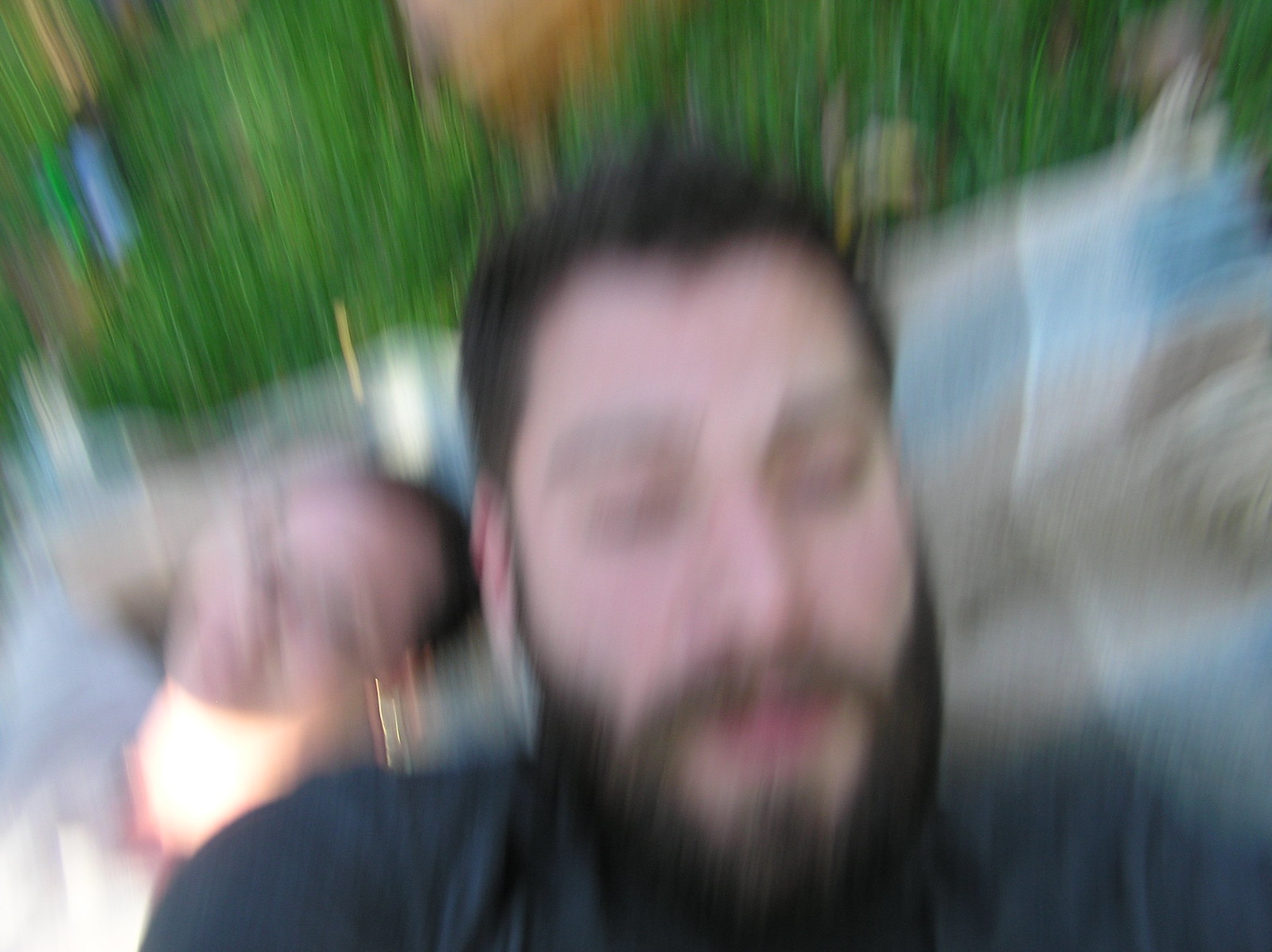A very blurry selfie photograph captures a man and a woman in an outdoor setting, possibly during a picnic. In the foreground is a man with a full beard and mustache, though the details of his facial features, including eyes and eye color, are indistinguishable due to the blurriness. His short hair, beard, and mustache are a dark brown color. Behind him, they appear to be lying on a blanket spread over the grass. The woman, positioned further back, has the sun reflecting off her neck, suggesting a bright day. She seems to be wearing eyeglasses, but, like the man, her features are too blurred to discern clearly. The overall color palette of the photograph consists of muted blues, greens, and grays, adding a soft, subdued feel to the image.